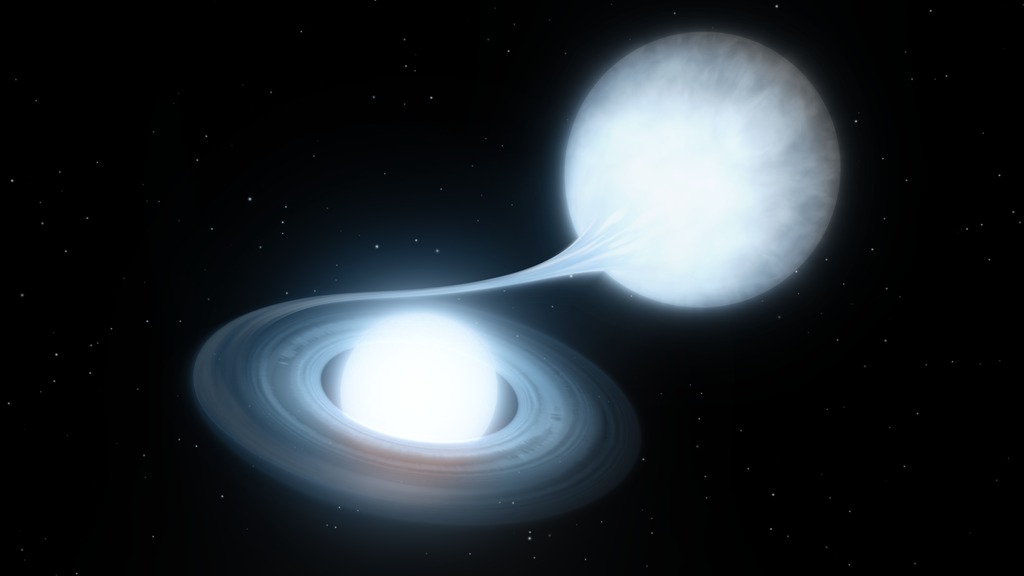This digital rendering vividly captures an outer space scene featuring a striking white planet situated prominently against a solid black sky, dotted with tiny white speckles representing distant stars. Central to the image is a dynamic swirl of colors—predominantly grays, blues, and subtle hints of brownish-red—emanating from the larger white planet. This swirl encircles and seems to envelop a smaller, luminously bright white orb, evocative of a moon or satellite. The artistic composition hints at the larger planet either consuming or drawing the smaller object into its vortex. The smaller orb is positioned in the top right quadrant of the image, while the larger swirling planet occupies the center and lower portions. There is no text overlay, allowing the mesmerizing visual elements to speak for themselves, creating a mysterious and captivating portrayal of a possibly cosmic phenomenon.